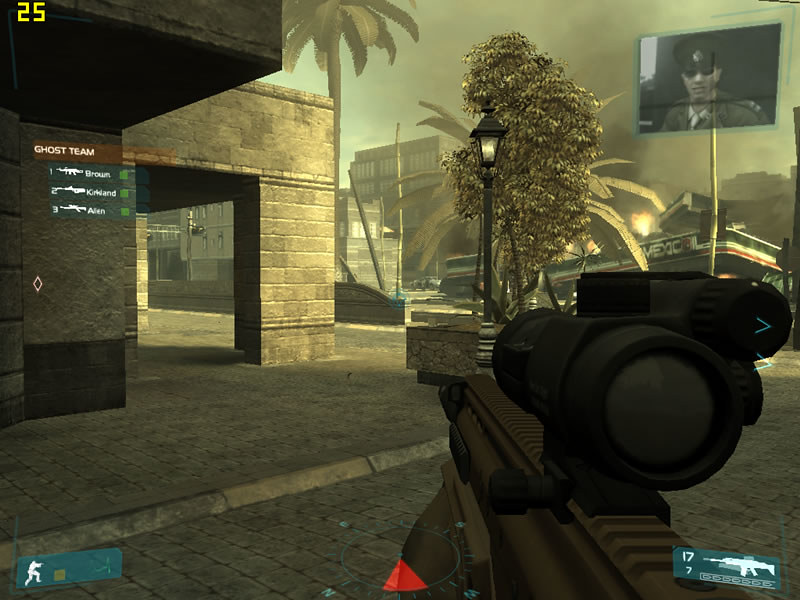This screenshot from a high-definition modern video game displays a highly detailed, immersive shooting environment. The vivid graphics present a post-apocalyptic scene with an array of tan and gray tones dominating the palette. From the first-person perspective, the player's character is wielding a black gun, ready for action. In the background, smoke rises, adding to the chaotic atmosphere. The setting features an architecturally distressed area with a brick building adorned with an arch on the left, and brick tiles underfoot. A curb is visible along the left edge of the frame, and some fire blazes in the background on the right side, further emphasizing the destruction. Notably, palm trees stand tall amidst the ruins. The interface includes yellow numerals "25" in the top left corner, likely indicating ammunition or health, and a small TV screen appears in the top right corner, possibly showing a mini-map or other crucial game information.